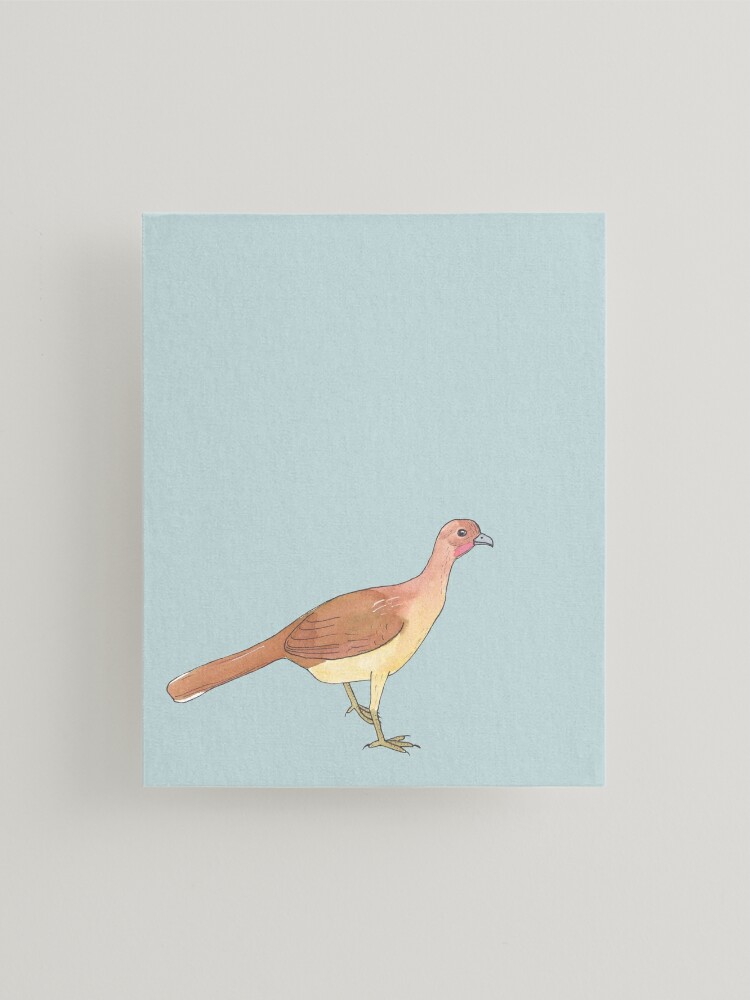The image features a vertically oriented photograph of a canvas hanging on a light gray, almost white wall. The canvas itself is a soft, robin's egg blue. At the center of the canvas, there is a watercolor painting of a bird, standing with its right side facing the viewer. The bird’s head and neck are tinged with a faded red hue, and it has a grey bill and a single, conspicuous black eye. Its underbelly transitions into a light peachy tan or orangish-yellow, while the side feathers and extending tail feathers are a delicate pastel brown. The tail feathers also have white lines along their edges. The bird is depicted with one foot on the ground and the other raised, suggesting motion. Additionally, its feet appear to be a light reddish-brown or green color. The depiction is somewhat childlike and rough in style, especially noted in the visible white lines around the feathers and the detailed yet simplistic rendering of the bird’s three-toed feet.